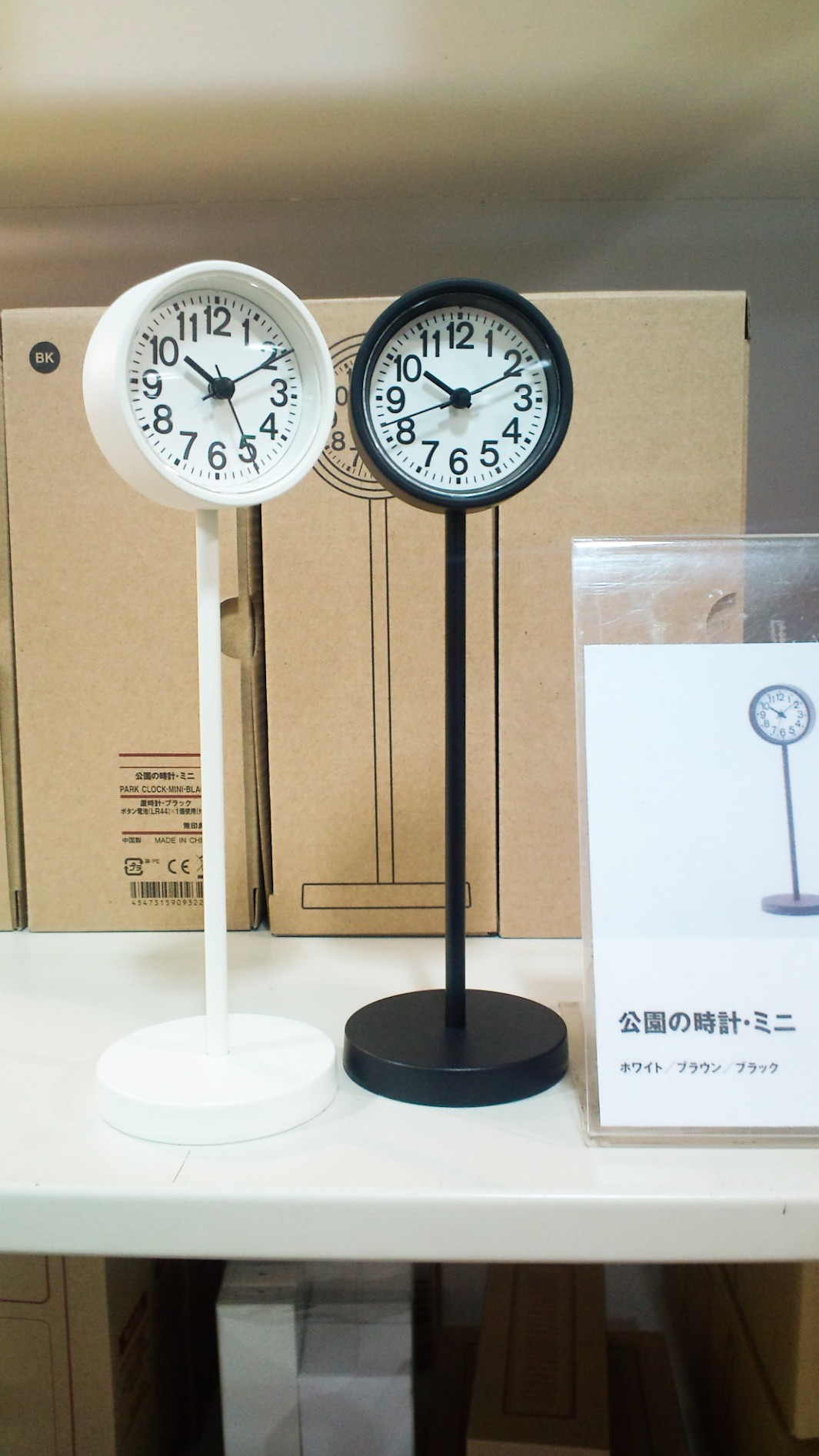In a store display, two clocks are prominently featured against a gray backdrop. They are placed on a pristine white table, with cardboard boxes arranged behind them. A Lucite holder stands between the clocks, containing a piece of paper with information about the clocks, though the text is in an unfamiliar language. 

What stands out about these timepieces is their unique design: each clock is affixed to a slender pole that culminates in a round base. Despite this unconventional mounting, the clocks themselves have a classic appearance with a standard 12-hour face, marked by numbers and minor ticks for the minutes. They also feature hour, minute, and second hands, although the second hands are not highlighted in red as is common. 

The clocks are identical in design save for their color - the one on the right is black while the one on the left is white. The white clock appears slightly larger, but this may be an optical illusion resulting from its position; it is placed slightly forward on the table and is angled a bit differently compared to the black clock.